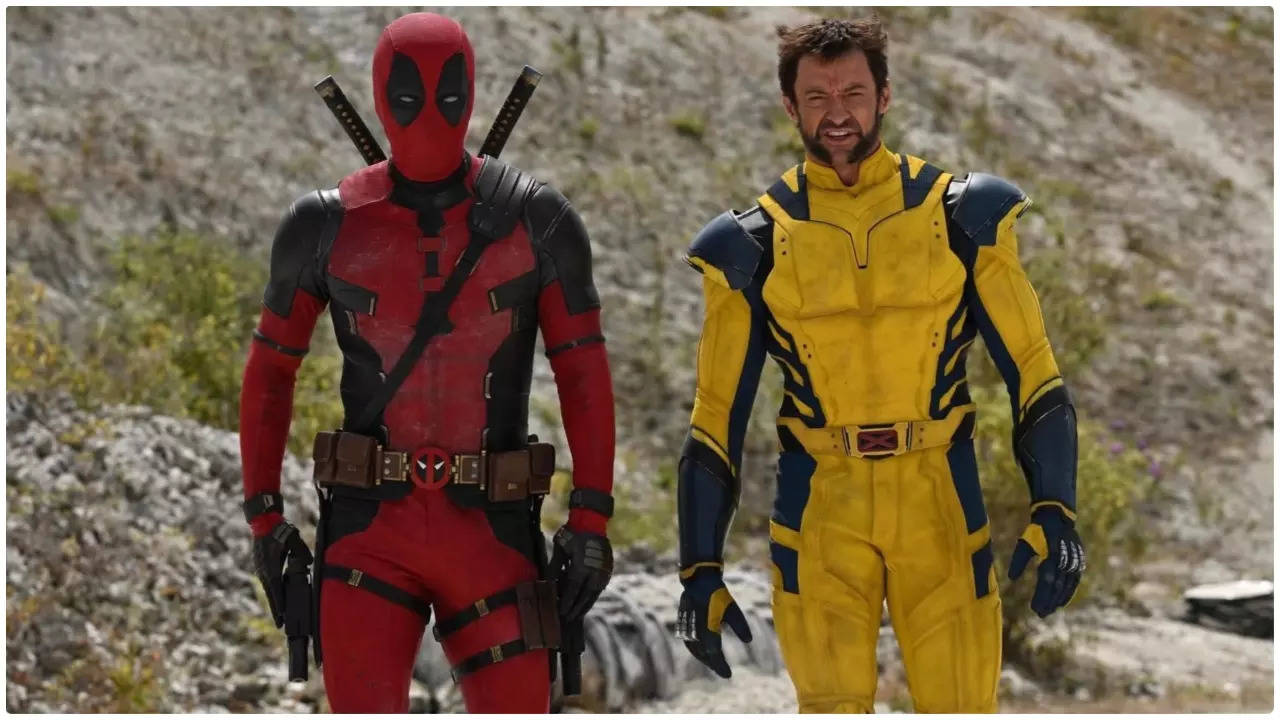The image captures a dynamic outdoor scene featuring two iconic Marvel characters, Deadpool and Wolverine, who appear ready for action. Deadpool, positioned on the left, is dressed in a striking red and black spandex outfit complete with black shoulder pads, gloves, a brown belt, and numerous weapons including guns in holsters and two swords strapped to his back. His face is visible, revealing a slightly open mouth, squinting eyes, and messy hair. To his right stands Wolverine, embodying Hugh Jackman's portrayal, clad in a distinctive yellow and black spandex uniform with black trim on the shoulder pads and gauntlets. Unlike Deadpool, Wolverine's costume lacks any headgear or visible weapons. The backdrop features a rocky, mountainous terrain dotted with green shrubs, under the bright daytime sun, suggesting a rugged battlefield environment.